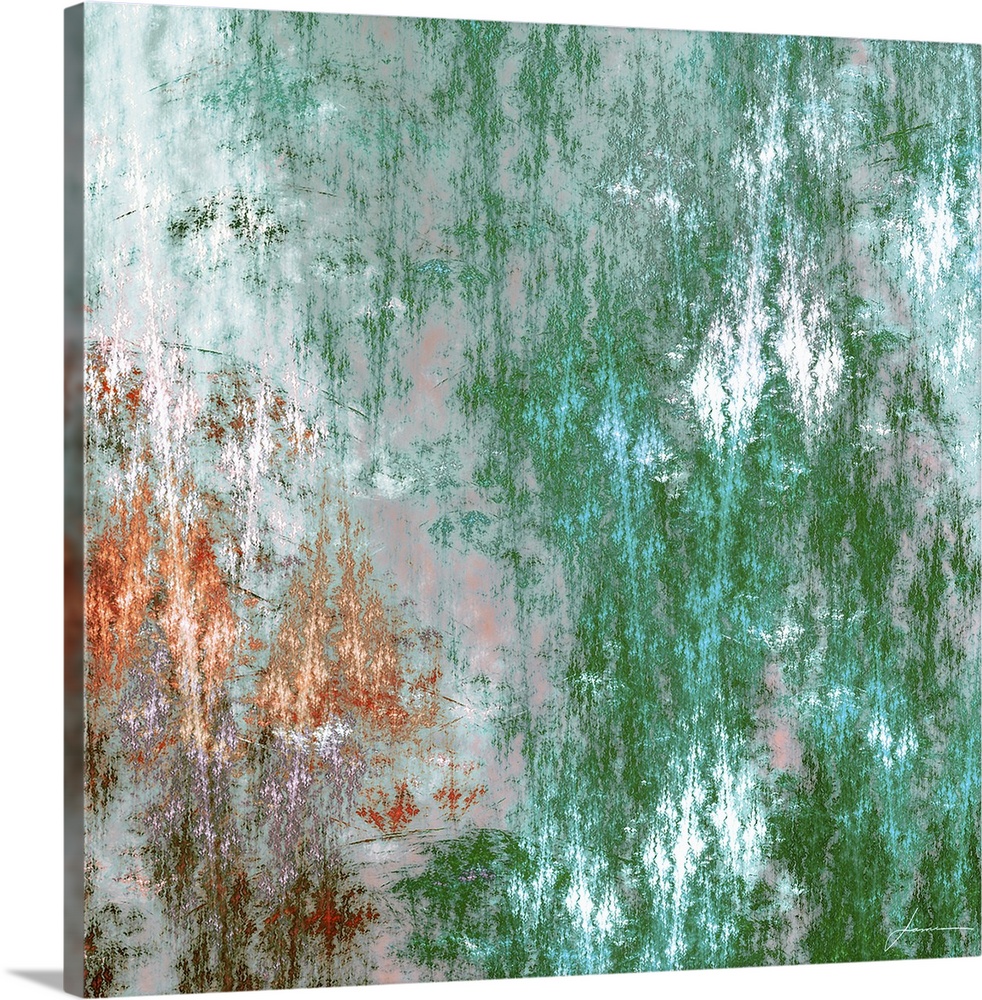The image resembles an impressionistic painting, primarily portrayed in green with copper hues. Dominating the right-hand side, tall green forms evoke a sense of pine trees emerging from a forest backdrop, suggesting a wintry day. On the left, a smaller section features copper-colored trees or bushes, adding a vibrant contrast. The painting's abstract nature and watercolor-like quality create a somewhat distorted appearance, making the exact details hard to discern. Overall, the colors blend harmoniously with hints of white, turquoise, red, and orange, enhancing its serene forest motif. In the bottom right corner, the artist’s signature, possibly "Johnson," is faintly visible, adding a personal touch to the artwork.